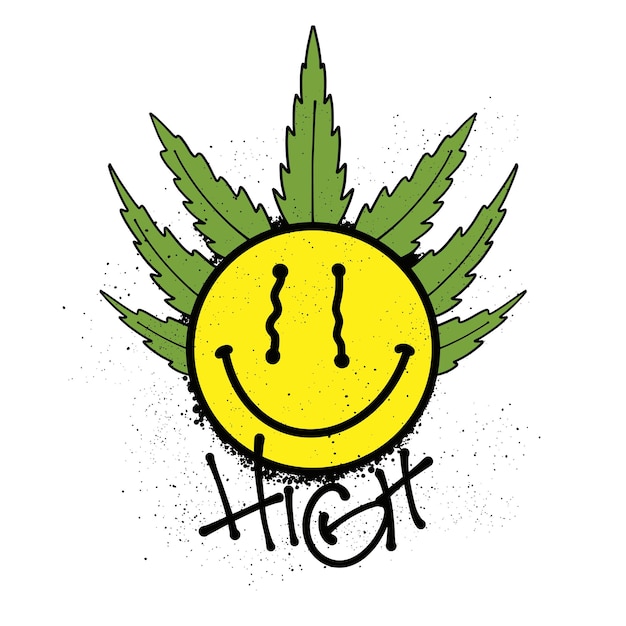This detailed digital drawing features a yellow smiley face with squiggly eyes and a semicircle smile at the very center, encased within a perfect black circle. Emanating from the top of the smiley face are seven green cannabis leaves, each sharply defined with black borders and central veins. Below the smiley face, the word "HIGH" is rendered in a graffiti style with thin black lines and surrounded by numerous black splatters, reinforcing the playful, edgy aesthetic. The entire image utilizes a limited color palette of green, black, yellow, and white, focusing on the contrast between these hues.